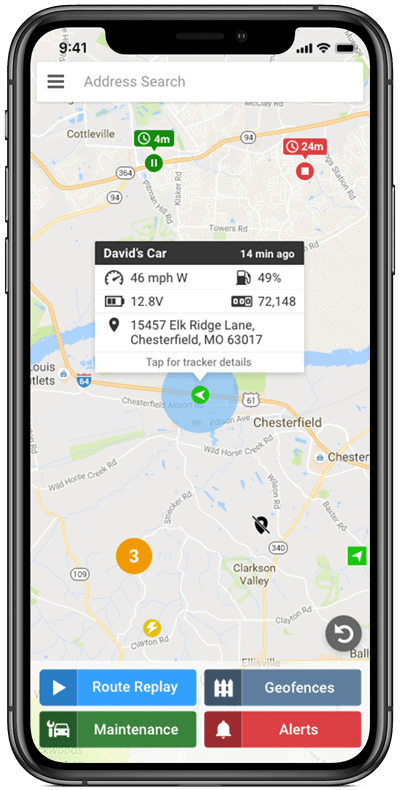This image depicts a smartphone screen displaying a detailed map interface for vehicle tracking. The phone's battery is fully charged, indicated by a black battery bar, and it has excellent connectivity with all signal bars full. The time displayed is 9:41 AM.

At the top of the screen, there's a white search box labeled "Address Search" with an icon of three horizontal bars next to it. The map shows the location of "David's car," which was last recorded 14 minutes ago. The information is highlighted in a black square and shows the vehicle traveling west at 46 miles per hour. The vehicle's battery level is at 12.8 volts and the gas tank is 49% full. 

An address, "15457 Elk Ridge Lane, Chesterfield, Montana," is listed, with a 5-digit number, "72148," possibly serving as an identifier. Another graphic presents a green circle with a leftward arrow in white, likely marking David's current position on the route.

The interstate on the map is highlighted in gold while other streets appear in white. Below the map, options are available for "Route Replay," "Maintenance," "Geofences," and "Alerts," each represented by red, green, gray, and blue boxes respectively.